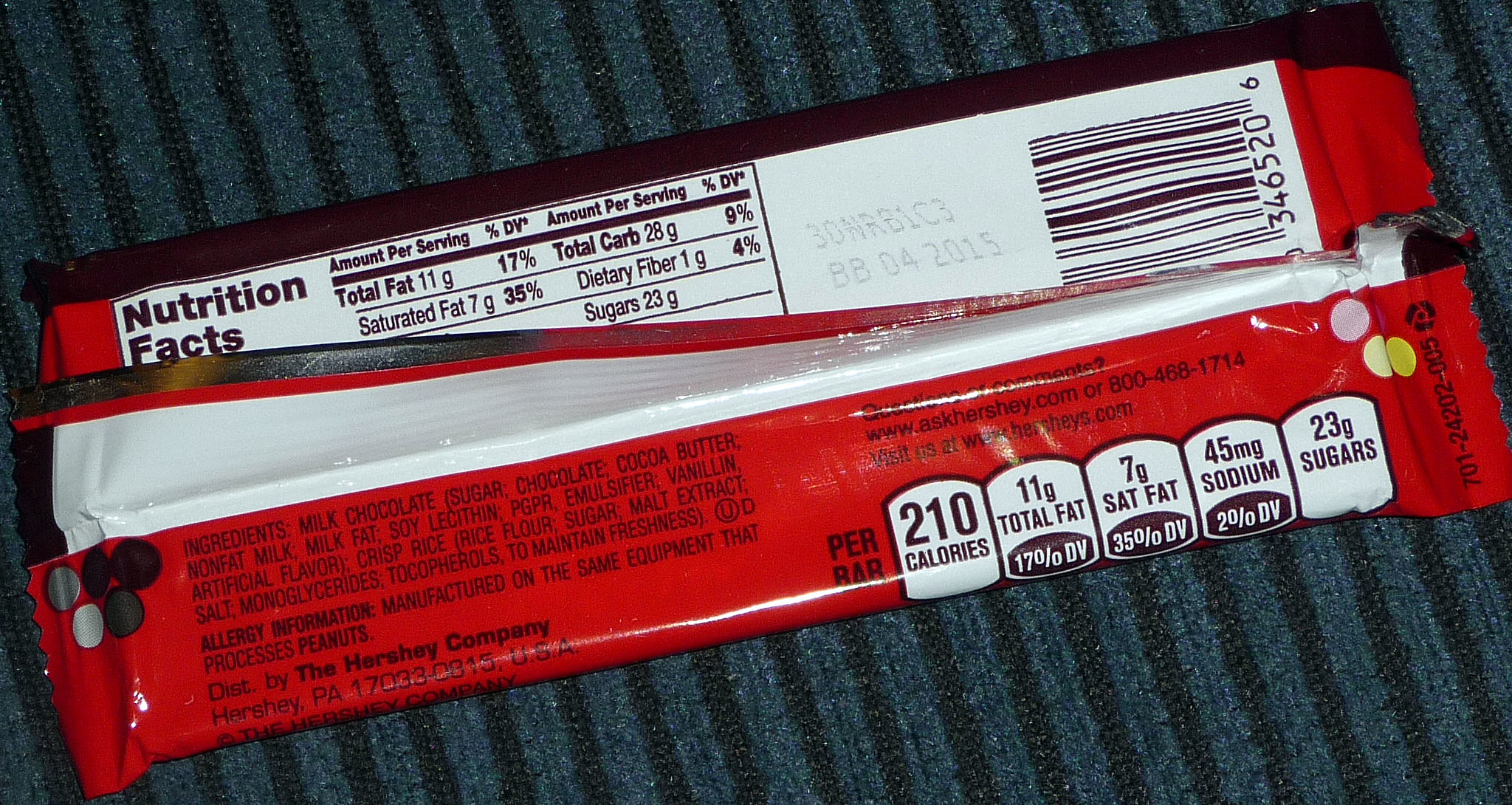On a vertically striped grayish-blue and gray fabric surface lies a partially opened or possibly empty candy bar wrapper. The wrapper is predominantly red with brown writing, and it is positioned upside down. The visible section of the wrapper prominently displays the nutrition facts and barcode at the top. The bottom portion reveals more detailed nutritional information along with the Hershey company branding. Additionally, there are two small dots—one pink and one yellow—on the right-hand side of the wrapper, adding a splash of color to the scene.